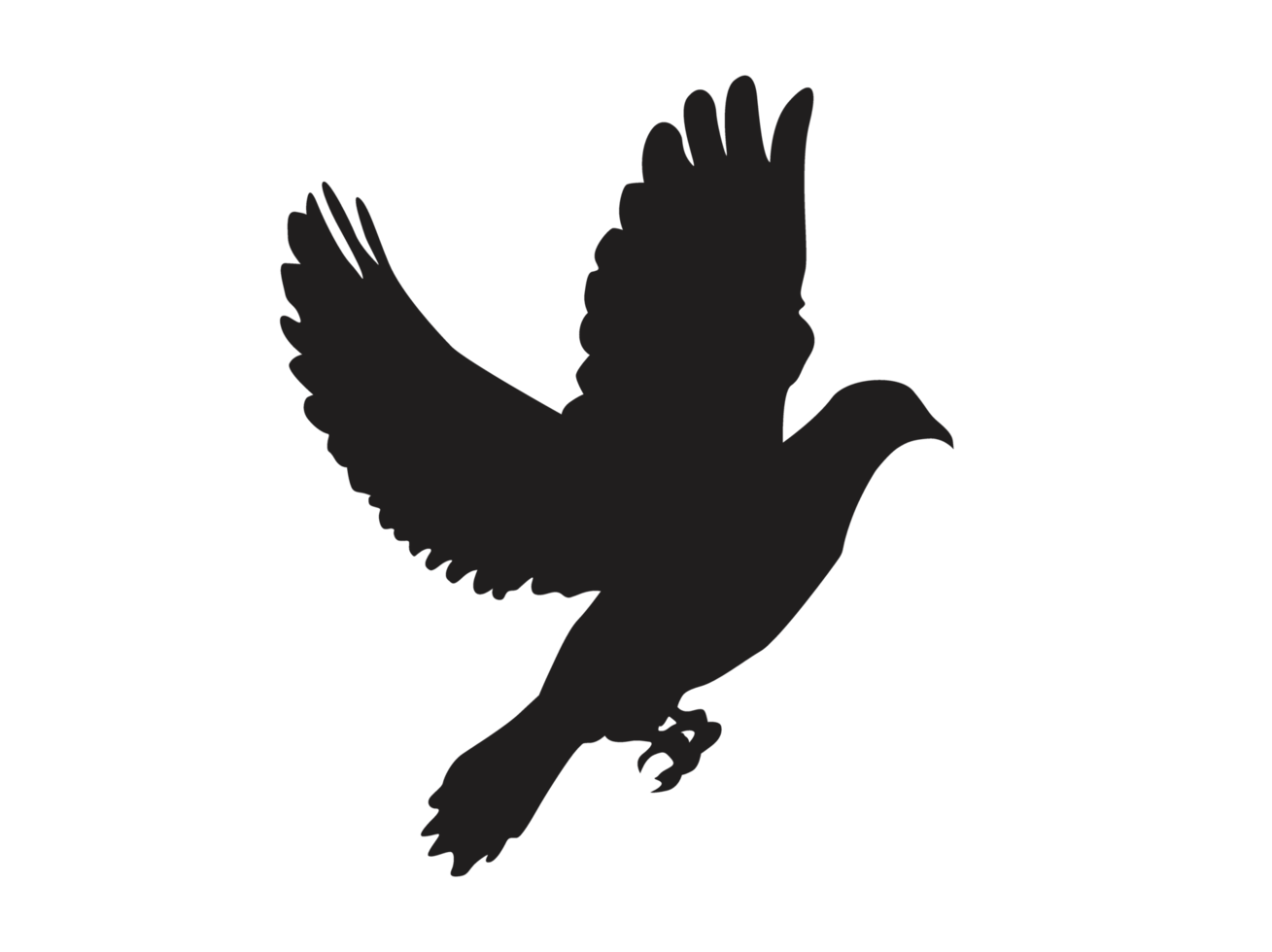The image depicts a large bird, fully rendered in a stark black silhouette against a plain white background. The bird, which could potentially be a bird of prey, a raven, a crow, or even a pigeon, is captured in mid-flight with its wings outstretched and its claws slightly curved as if anticipating a perch. The beak, visible with a subtle downward curve, hints at a possibility of it being a raptor. The detailed outline showcases the individual feathers on both wings and the entire body, emphasizing its looming, almost majestic presence. The bird's orientation is towards the right, with its tail and each talon clearly discernible, creating a simple yet striking image reminiscent of classic Victorian silhouettes, embodying both grace and anticipation.